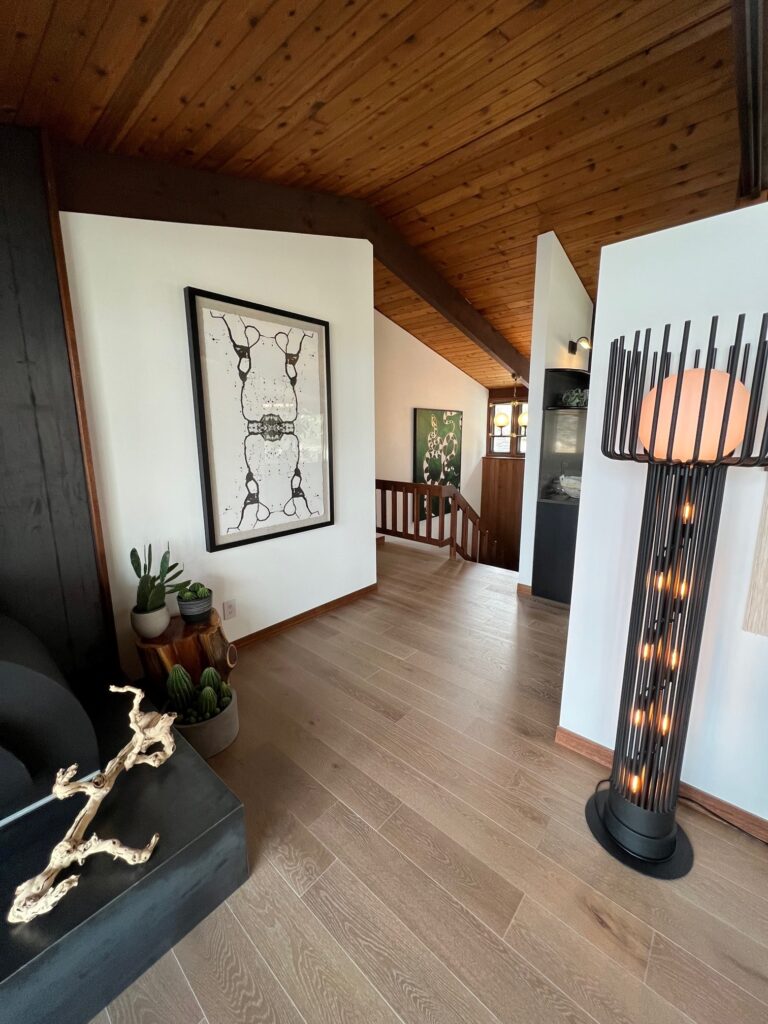This indoor daytime photograph captures an elegantly designed modern space. The room features a clean, light brown hardwood floor juxtaposed against a combination of white and dark wood walls. A black-framed piece of abstract art with a green background and possible snake imagery adorns the white wall. To the right side of the image, there's a black, modern, cylindrical lamp with small light bulbs spiraling up its base and a larger circular bulb at the top. Additionally, a unique statue that incorporates a ball element adds to the modern art vibe of the room. A wooden ceiling with exposed beams supports two lit lights attached to a central beam. On the left, a tree trunk-shaped wooden end table holds an arrangement of small cactuses and succulents, which may be artificial. The room also includes a wooden railing and a set of stairs leading down to a lower level, contributing to the open and spacious feel of the interior design.